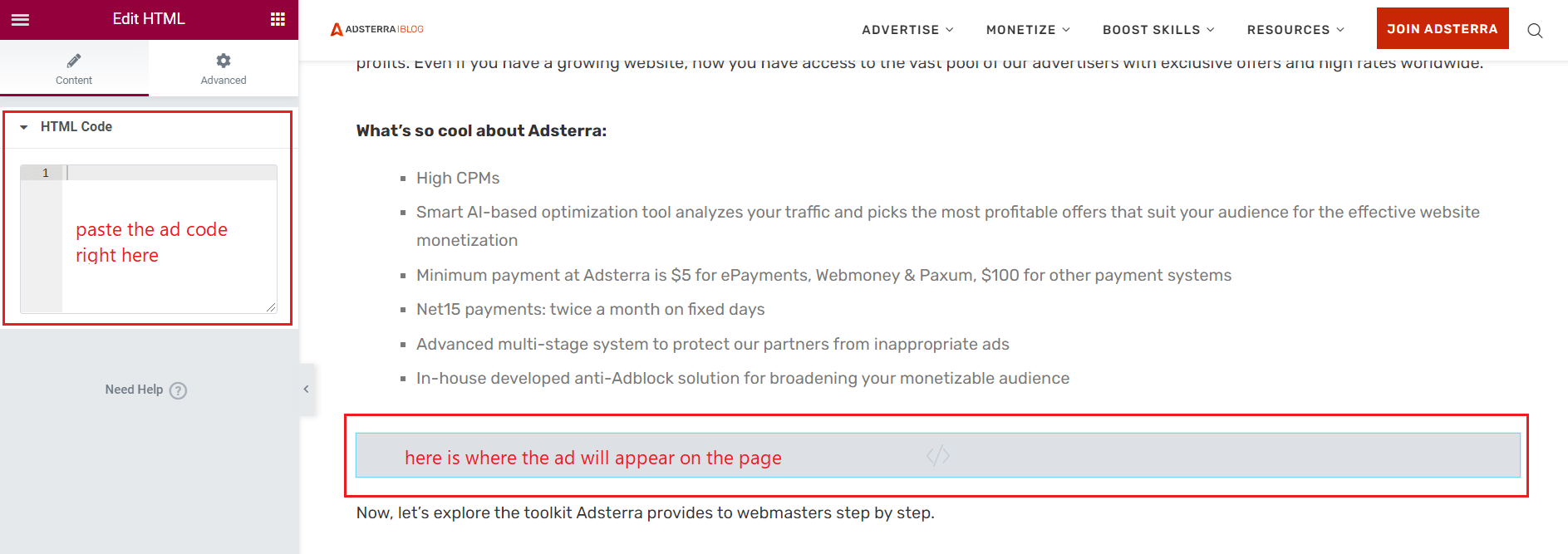The image depicts a detailed screenshot of a website's editing interface, along with various content sections and navigational elements.

On the left side of the screen, there is a vertical panel framed in reddish-purple at the top, labeled "Edit HTML." This section includes a drop-down menu indicated by a three-lines icon to the left and a grid icon featuring three rows and columns of squares on the right. Below this border, two tabs are visible: "Content," marked with a pencil icon, and "Advanced," represented by a settings gear icon. Underneath these tabs, there is a section labeled "HTML code." Within this section, there is a text insertion box bordered in gray, with red text inside the box instructing users to "Paste the ad code right here." This box is outlined by a red rectangle. Further down, there is a gray rectangular panel that reads "Need help," accompanied by a gray question mark icon.

On the right side, the main content area features a white background. At the top, a logo on the left displays the word "Adtera" next to a red triangular symbol, possibly indicating this is a blog. To the right of the logo, a black navigation menu lists the options "Advertise," "Monetize," "Boost skills," "Resources," each followed by a downward carrot icon. Additionally, there is an orange button labeled "Join Adtera" and a magnifying glass icon representing the search function.

The main content area also includes a section where the page has already scrolled down, making the top header partly unreadable. Below this, a visible heading in black reads "What's so cool about Adtera." This is followed by a bullet point list in dark gray font that highlights features like:
- High CPM rates.
- A Smart AI-based optimization tool for monetizing websites effectively.
- A minimum payment threshold of $5 for e-payments and $100 for other systems.
- Net 15 payments, made twice a month.
- Advanced multi-stage systems for ad protection.
- An in-house anti-ad block solution to expand the monetizable audience.

Further down, a long, skinny horizontal gray border outlines an area in red that states, "here is where the ad will appear on the page." Below this, in small black font, it reads, "Now let's explore the toolkit Adtera provides to webmasters step-by-step.”